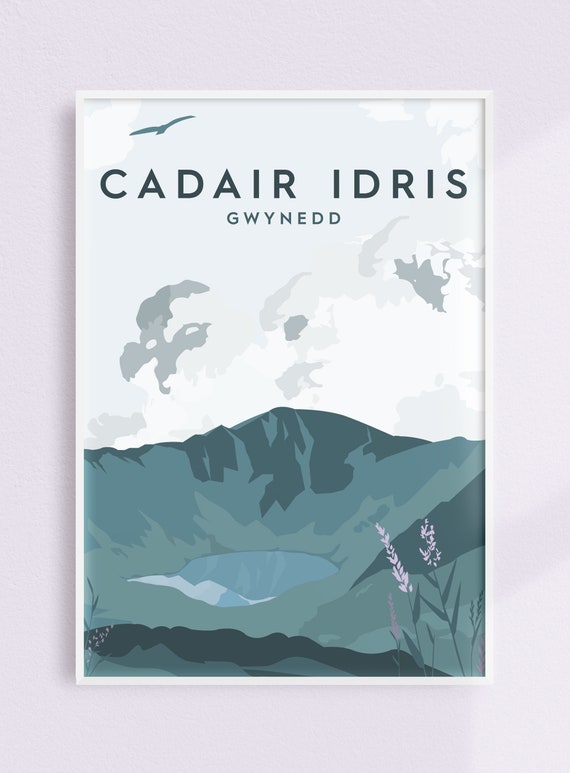Framed in a thin, white frame and hung on a vivid pink wall, the artwork presents a stylized, almost impressionistic scene. At the top of the piece, the text "CADAIR IDRIS GWYNEDD" stands out in large, bold, black capital letters. Above the text, a blue bird is seen flying in the top left corner, adding a touch of liveliness to the sky. The sky itself transitions from shades of mint green to white and gray, with clouds that some describe as resembling country outlines on a map.

Beneath the text, the landscape unfolds into a serene mountain scene. The mountains are depicted in a palette of dark blue, turquoise, and green shades, forming a canyon area with an inviting lake nestled in the middle. This lake, surrounded by the rugged mountain terrain, appears to be a serene pool of water, possibly with hints of snow. In the bottom right corner of the image, delicate pink flowers emerge, adding a splash of color to the predominantly cool-toned artwork. Overall, the piece evokes a tranquil yet majestic natural landscape, framed beautifully against the contrasting pink wall.